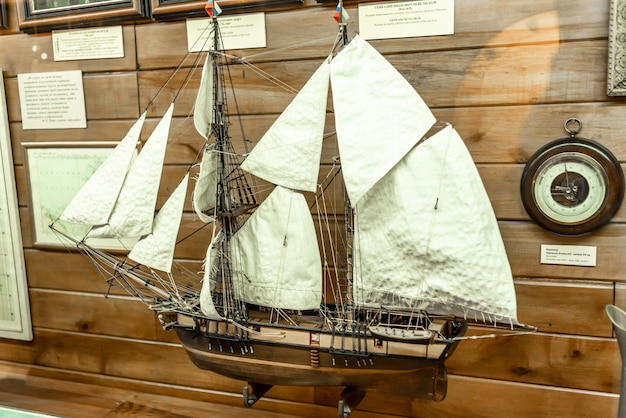An impressive handcrafted wooden model ship with nine billowing white sails stands proudly on display against a warm brown wood-paneled wall in what appears to be a nautical museum exhibit or gallery. The ship's sails are meticulously detailed and connected by intricate rigging, emphasizing the model's precision craftsmanship. Adorned with little red, blue, white, and gray flags atop its two masts, the ship exudes a sense of historical significance. Surrounding the ship on the wall are various nautical artifacts, including what seems to be a compass with a brown outer rim and another measuring device, each accompanied by small informational plaques. Although the text on these plaques is too small to be legible, their presence underscores the exhibit's educational intent. A potential sun glare or reflection in the upper right-hand corner suggests that the model is showcased within a glass case, further enhancing its prominence in this thoughtfully arranged display.